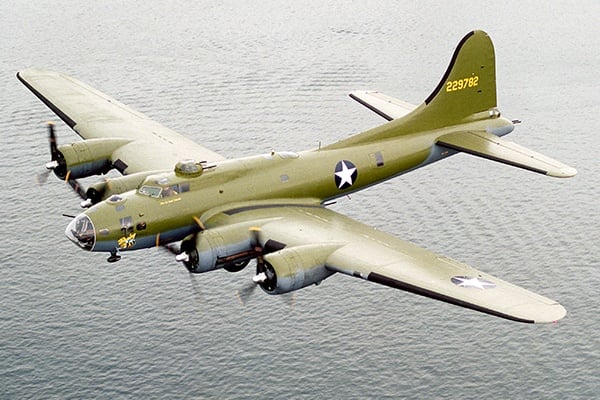The image captures an overhead view of a World War II fighter-bomber aircraft flying over a vast ocean. The plane is large and distinctively painted in army green on the top and silver on the bottom. Prominent white stars set within a blue circle adorn the sides and wings of the aircraft, symbolizing its American origin. The back tail of the plane, rounded and prominently marked, bears the yellow number 229782. Each wing hosts two of the plane’s four propellers, visible along the front wings close to the cockpit area. The front nose of the aircraft is clear and likely designed as a shooting cone for military purposes, while the central cockpit turret is equipped with twin machine guns. The overall sleek and powerful design unmistakably identifies it as a World War II era fighter jet, gliding smoothly above the expansive waters below.